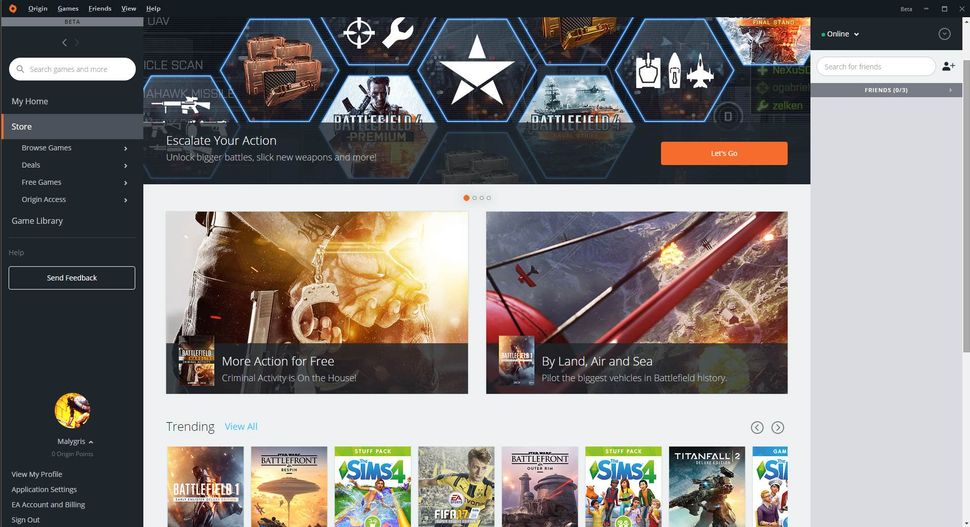This image depicts the homepage of a black-themed gaming website interface, likely associated with Origin by EA. In the upper left corner, there is an orange square with a black circle inside it, representing the Origin logo. Adjacent to this are menu options labeled "Games," "Friends," "View," and "Help." On the upper right, there are standard window control buttons: minimize, maximize, and close.

A black navigation band with white lettering is located on the left side of the screen. Below the navigation bar, there is a "BETA" tag. The navigation options include "Home," "Store," "Browse Games," "Deals," "Free Games," "Origin Access," "Game Library," "Help," and a "Send Feedback" button. There's also a search bar labeled "Search games and more," situated in white against the black background.

The user is on the "Store" tab, where the main content features a series of images arranged in a honeycomb-like hexagonal grid. Below the hexagonal images, a promotional banner reads "Elevate your action, unlock bigger battles, new weapons and more." Further down, there are several game images, including two prominent ones followed by a series of smaller images, suggesting the presence of a carousel for browsing featured games.